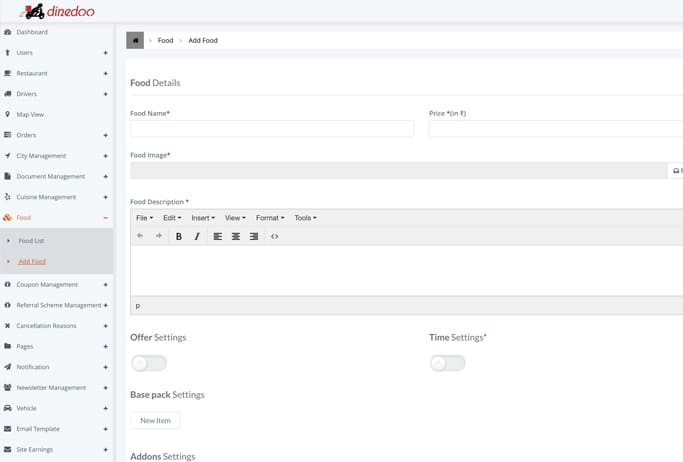This is a detailed screenshot of a desktop interface for the "Dine & Do" application. In the upper left-hand corner, a distinctive logo featuring a motorcycle rider zipping forward is displayed, with the brand name "Dine & Do" written in red lowercase letters next to it.

Below the logo, a vertical menu provides various management options. The menu items listed are:

- Dashboard
- Users
- Restaurant
- Drivers
- Map View
- Orders
- City Management
- Document Management
- Cuisine Management
- Food (highlighted with a dropdown showing "Food", "Line", "Add Food")
- Coupon Management
- Referral
- Scheme Management
- Cancellation Reasons
- Pages
- Notification
- Newsletter Management
- Vehicle
- Email Template
- Site Earnings

Most of these menu items have a plus sign on the right-hand side, indicating that more filters or options can be dropped down.

At the top of the main content area, a banner indicates that the "Food" section is open and "Add Food" has been selected. Below this, the interface for adding a new food item is visible, which includes fields for "Food Details" such as:

- Food Name
- Price
- Food Image
- Food Description

Additional settings include toggle buttons for "Offer Settings" and "Time Settings". The section also includes options for "Base Pack Settings", with a button to "Add New Item". The screen is cut off at the bottom, but you can partially see the "Add-On Settings" section.

This comprehensive interface provides a detailed and organized way to manage various aspects of the "Dine & Do" food delivery application.